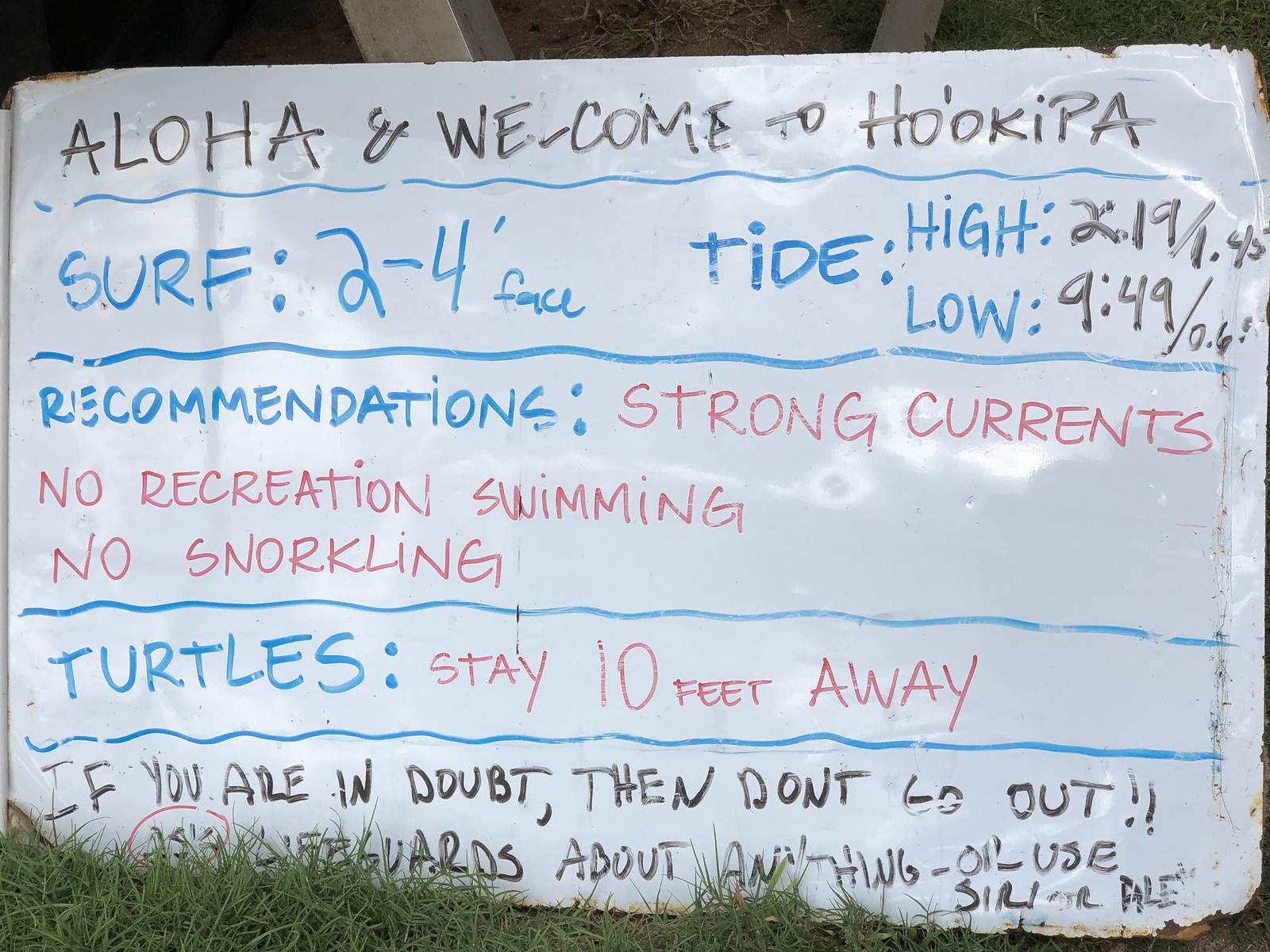The image depicts a vertical dry erase board situated on a bed of grass, reflecting a lot of light. The board is propped against a 2x4 and has various instructions written in multiple colors of markers. At the top in black marker, it reads, "Aloha and welcome to Ho‘okipa." Below that, a blue dividing line separates the header from the main content. In blue marker, the board lists surf conditions: "Surf: 2-4 feet face, Tide: High 2:19, Low 9:49." Another blue dividing line follows, leading to recommendations in blue marker. In red marker, it warns about strong currents, and advises "No recreational swimming" and "No snorkeling." After yet another blue dividing line, the word "Turtles" appears in blue, followed by a red caution to "Stay 10 feet away." At the bottom, in black marker, it cautions, "If you are in doubt, then don't go out," and advises to ask lifeguards about anything. Some letters at the bottom are obscured by grass, and certain parts appear partially erased.